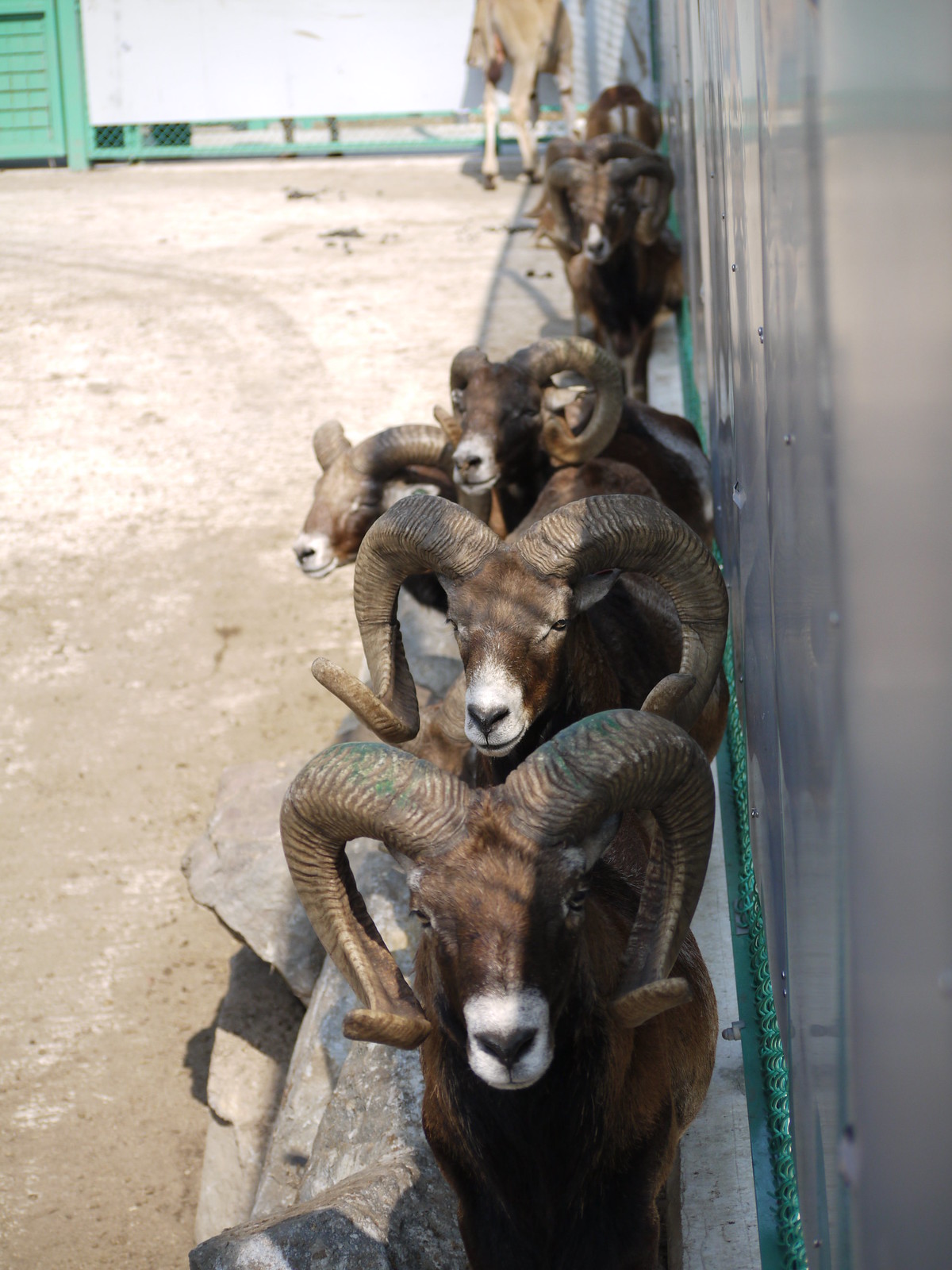The photograph captures a detailed and striking scene of six bighorn sheep standing in a neat row, all with their characteristically large, curved horns. These sheep have distinctive features: their bodies are a rich brown, contrasting with the white patches on their faces and the black tips of their noses. They are huddled closely against a metallic silver wall, which could be part of a pen or a metal vehicle, seeking the last bits of shade as the sun encroaches. The ground beneath them is barren dirt, and a green rope runs parallel to the wall, hinting at additional enclosure boundaries. Off in the distant background, there seems to be another tall animal with a black-tipped tail, possibly a young camel. A green fence can also be seen in the back left corner, completing the enclosure scene. The alignment and attentive stances of the sheep make for a captivating, orderly composition.